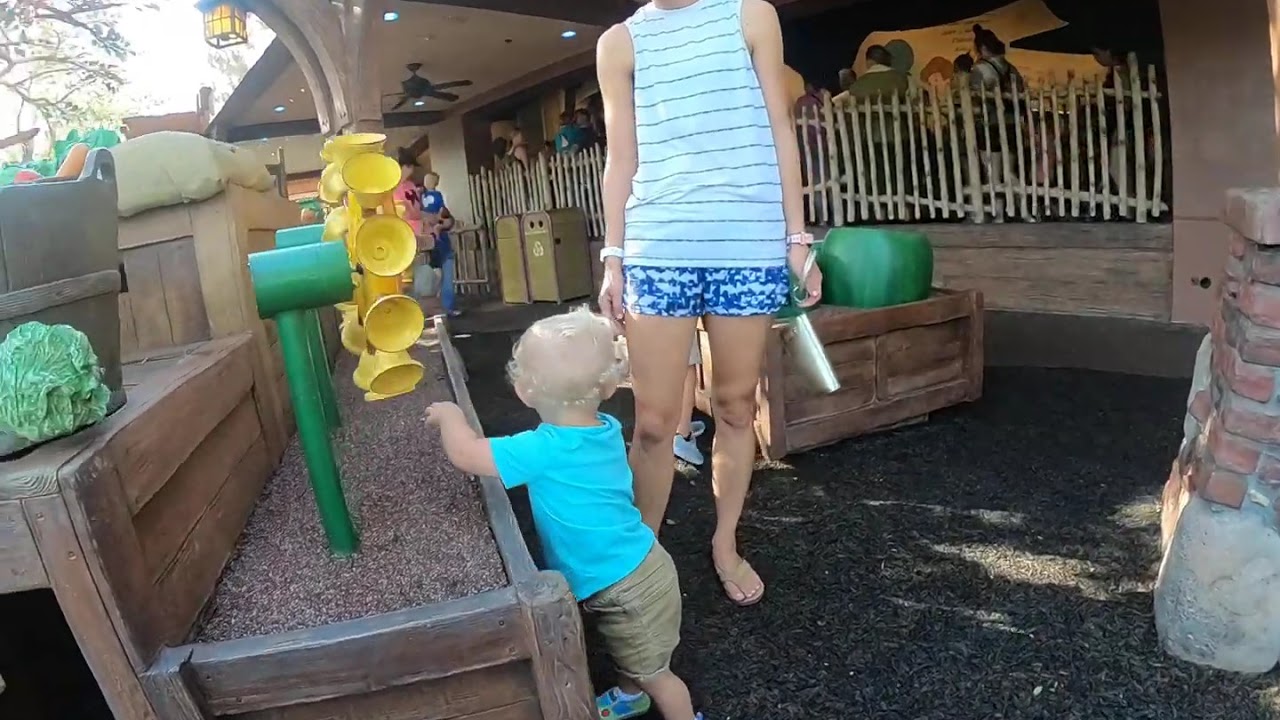In this outdoor daytime scene, a toddler, likely around two years old, with blonde hair, is standing in a play area. The child is dressed in a blue shirt and beige shorts. Nearby, a woman, possibly the child’s mother or babysitter, is positioned behind the toddler, wearing a white striped tank top paired with blue shorts. She holds an object in her left hand, possibly a purse. The play area features various elements including a toy with yellow horns, a wooden picket fence, raised wooden beds with shredded rubber tire mulch, and scattered bricks. In the background, more children can be seen enjoying the play area while a few adults are gathered behind the fence. The area also contains yard elements such as a tree, sheds, pots, and perhaps a barbecue setup, suggesting this could be a public recreation spot or an amusement park environment. The vibrant colors present include shades of blue, aqua, green, and yellow, adding to the lively atmosphere of the scene.